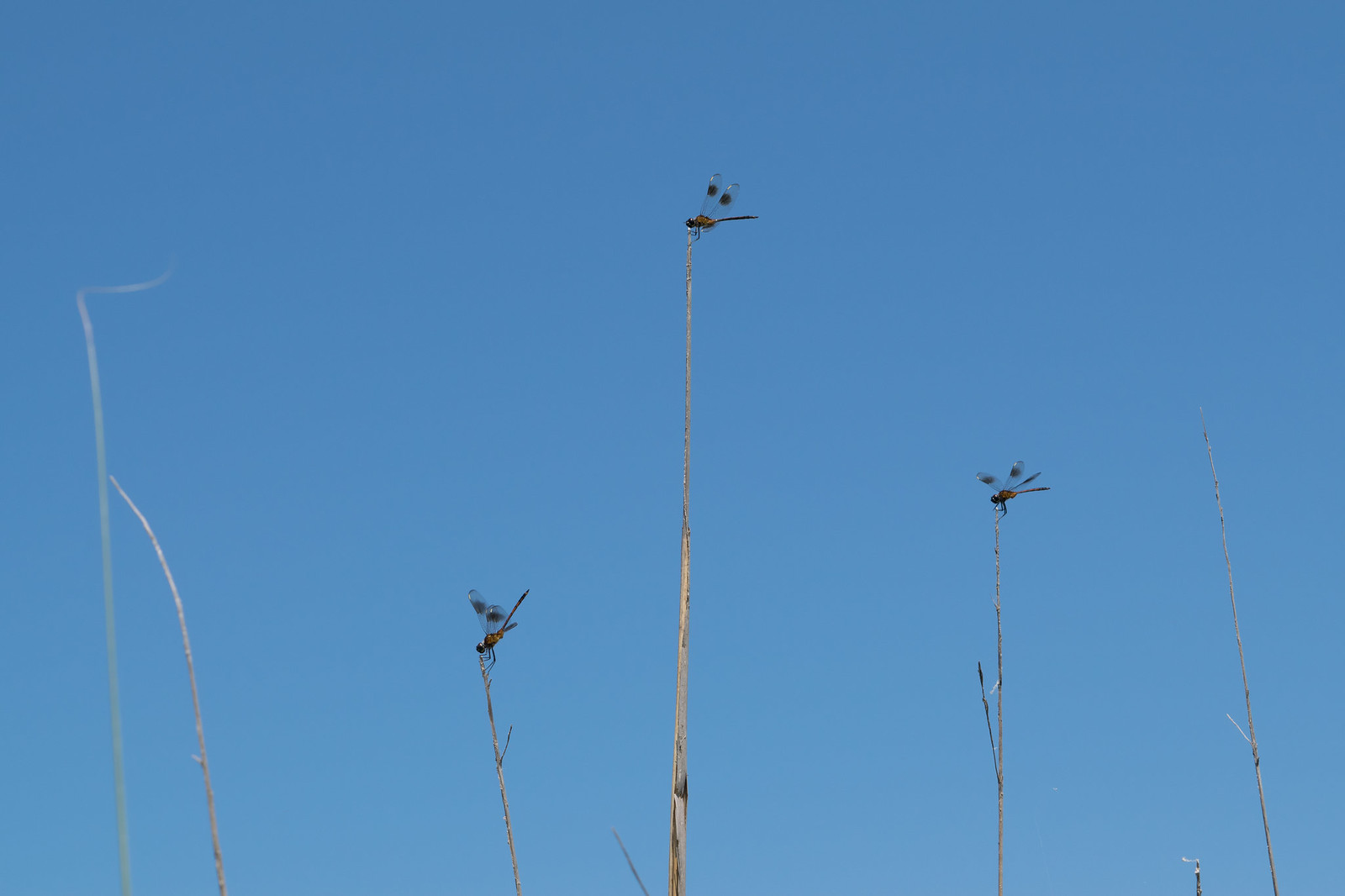This is a color photograph capturing a bright blue sky that occupies nearly the entire frame, devoid of any clouds, suggesting it was taken in the clear, midday light. Dominating the scene are five tall, slender metal poles, resembling either electricity or lighting poles, clustered towards the center and right of the image. The leftmost pole is distinctive, branching into two parts near its base. Three of the central poles feature tiny red ledges and spikes at their tops. Perched atop these poles are several birds: two on the first and the middle poles, and two more on the next pole to the right. Additionally, there are very thin branches or straw-like structures in the foreground, some standing upright with clear and black-spotted leaves. One central blade of straw stands out at about six inches tall, with delicate black leaves and two clear leaves tipped with black circles. Within these branches, there are small insects with brown bodies and long, clear wings lined with silver, some in a state of motion evidenced by their blurred outlines. The detailed interplay of elements against the expansive sky creates a dynamic yet serene composition.